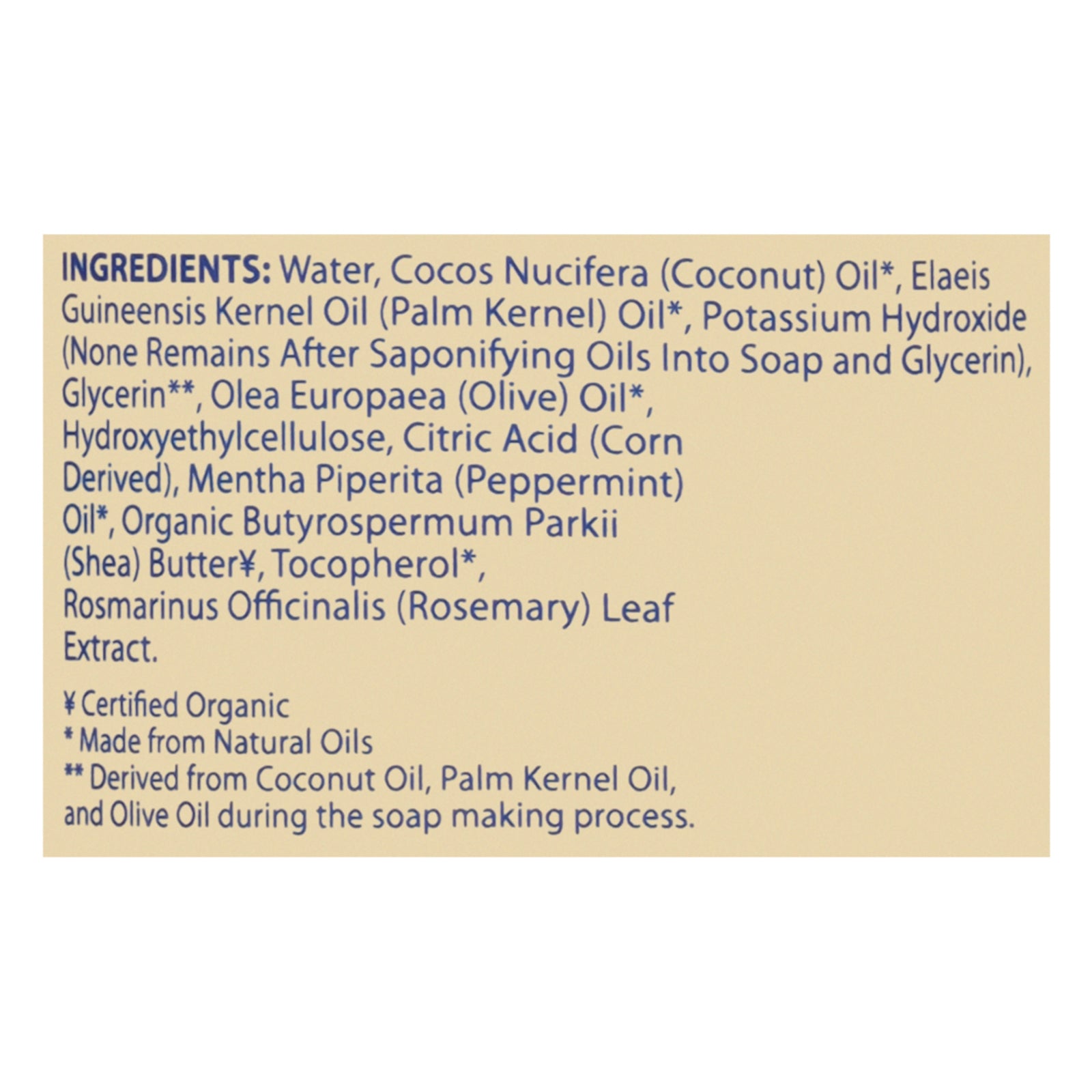The image is a horizontal rectangular photograph of an ingredients label on a product. The label has an off-white, tannish background with bold blue text at the top that reads "Ingredients:" followed by a list of the ingredients in non-bold blue text. The ingredients listed are: water, cocos nucifera (coconut) oil, elaeis guineensis (palm kernel) oil, potassium hydroxide (none remains after saponifying oils into soap and glycerin), glycerin, olea europaea (olive) oil, hydroxyethyl cellulose, citric acid (corn-derived), mentha piperita (peppermint) oil, butyrospermum parkii (shea butter), tocopherol, and rosmarinus officinalis (rosemary leaf extract). At the bottom of the label, there are several symbols and lines of text. One symbol resembles a letter "Y" with two lines through it, indicating "Certified Organic." Below that, there are notes marked by asterisks explaining that the product is made from natural oils derived from coconut oil, palm kernel oil, and olive oil during the soap-making process.